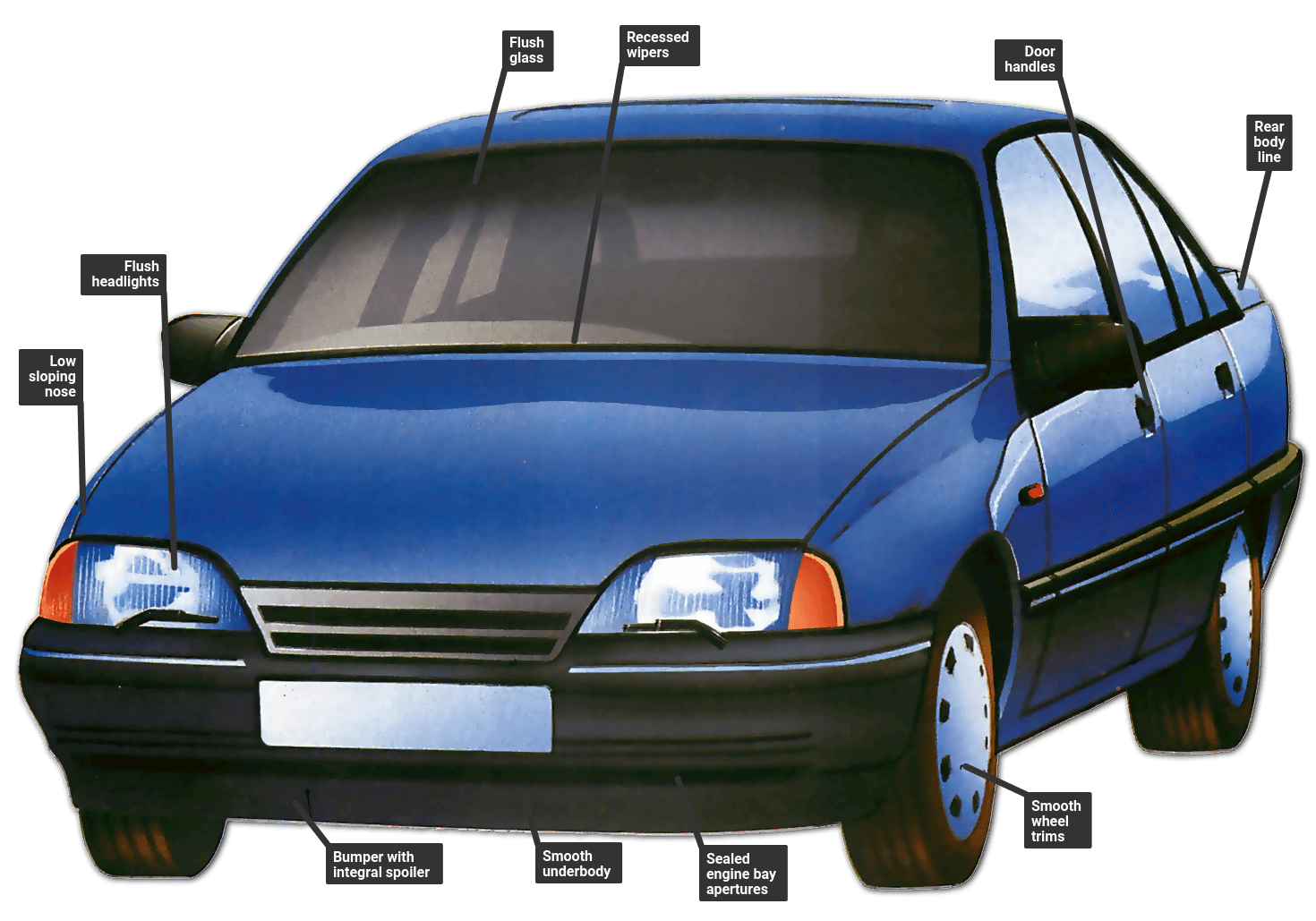The image is an informational chart showing a detailed 2D illustration of a blue, four-door compact sedan, devoid of any manufacturer identifiers. The car is comprehensively labeled with various features. Starting from the top left, a black box labeled "flush glass" points to the windshield, followed by "recessed wipers" indicating the area below the windshield. Continuing right, "door handles" points directly to the car’s door handles and "rear body line" aims towards the trunk. 

Along the bottom of the image, labels also follow from left to right. "Smooth wheel trims" points to the hubcaps, "sealed engine bay apertures" directs attention to the grille, "smooth underbody" indicates underneath the car, and "bumper with integral spoiler" highlights the bumper. The tires are partially depicted with an orange hue. Despite all the detailed labeling of features, the car lacks any license plates. The black rectangular boxes with white text clearly explain each pointed feature, making this a highly informative and detailed visual aid for understanding the car’s design elements.